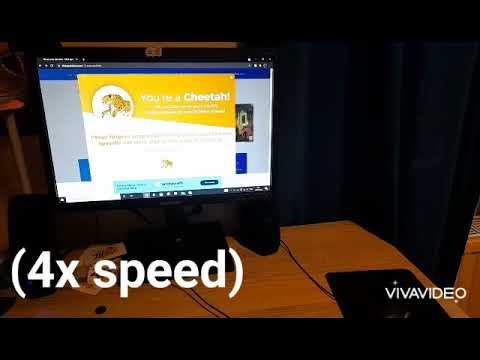In this image, we see a computer monitor with a sleek black frame, positioned on a light tan wooden desk. A pair of small black speakers flank each side of the monitor, which is displaying an online window. Although the resolution is low, the window features a prominent pop-up with a yellow background. On the left side of the pop-up, there is a white circle containing a cartoon depiction of a yellow cheetah. The text within the pop-up, in big white letters, reads "You're a cheetah." Below this message, in white parentheses, it states "4x speed." Further details include a black keyboard and a black mouse on a mouse pad situated to the right of the computer. The words "VIVA VIDEO" appear in all capitals at the bottom right corner of the screen. In the background, there's a heavy blue drape, adding a sense of depth to the scene. The image is slightly dark, suggesting the photo was taken in a dimly lit room.